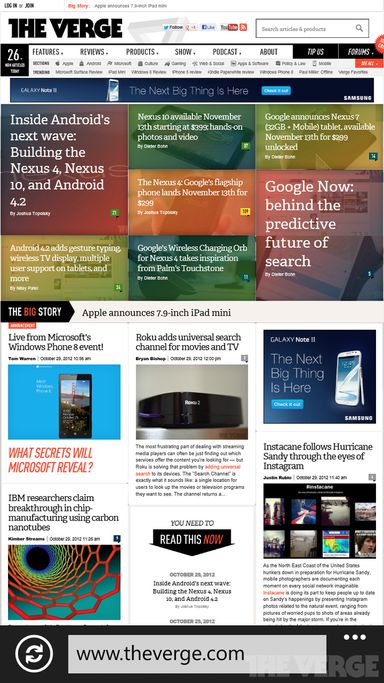Screenshot of The Verge website displayed on a smartphone in desktop mode. The dense layout is compressed into the vertical screen, reflecting an older version of the tech website. The address bar is located at the bottom of the browser, although the specific browser is not identifiable. A Verge watermark is visible in the bottom right corner of the screenshot. The main section showcases a variety of tech-related articles, such as "Inside Android's Next Wave," "Google Now: Behind the Predictive Feature Search," and topics on carbon nanotubes and Hurricane Sandy. The site features a prominent white background with vibrant colors used in the fonts and article backgrounds. Key website subsections are listed at the top right: Features, Reviews, Products, Show, Podcasts, and About.